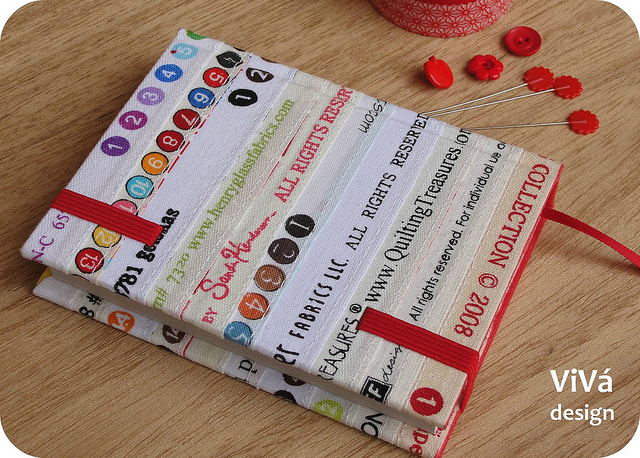The photograph, a rectangular image with rounded corners, showcases a handmade book cover lying on a light-grained, brown wooden table with a clear wood grain pattern running diagonally from the lower left to the upper right. The book cover, designed by Viva Design, prominently features its logo, "VIVA," in white text at the bottom right corner. The cover is an eclectic patchwork of fabric scraps, creatively repurposed from the selvage edges of different textiles. These scraps are characterized by circles filled with various colors like red, blue, dark red, orange, light blue, pink, yellow, purple, magenta, and green, each marked with corresponding numbers ranging from 1 to 10. 

Additionally, the book is secured with a red stretchy band and includes a red ribbon to mark the reader's place. Surrounding this artistic centerpiece are details such as small metal rods shaped like flowers, a small red bowl, and decorative elements like bobby pins with red handles and three red buttons—one shaped like an apple, another like a flower, and a simple red circle. A scroll of red lace adds to the overall vibrant and intricate composition, highlighting the meticulous and creative effort put into the design.